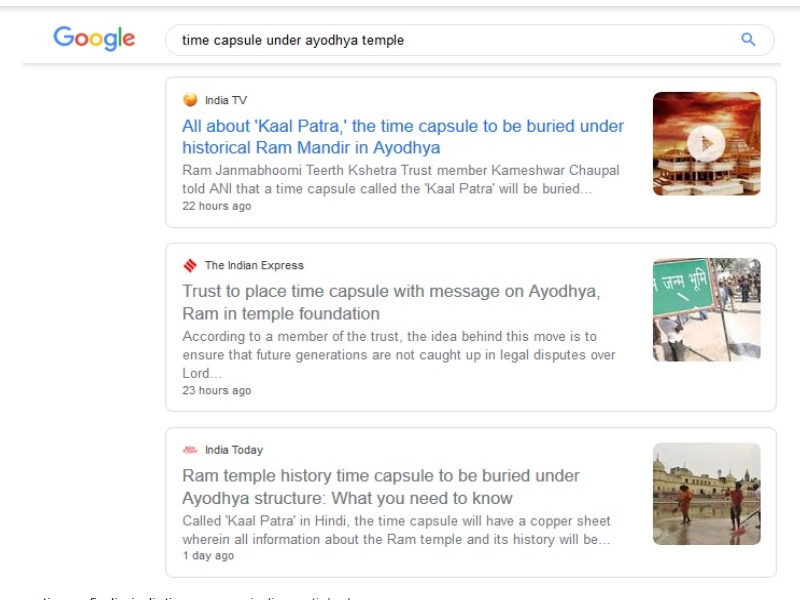This image is a screenshot of a Google search page. At the very top, there is a thin gray horizontal bar with a slight gradient effect. Below this bar, the Google logo, featuring its iconic colored letters, is prominently displayed. Centered under the logo is the search bar, which contains the search query "time capsule under Ayodhya temple."

Underneath the search bar, there is another thin gray bar similar to the one at the top but it does not span the entire width of the page.

Below this second gray bar, the top search results are displayed, each marked as a news article:

1. The first result, from India TV, is titled "All about Kalpataru: The Time Capsule to Be Buried Under Historical Ram Mandir in Ayodhya." It states that Ram Janmabhoomi Teerth Kshetra Trust member Kameshwar Chowpole informed ANI that a time capsule called the Kalpataru will be buried. This result was published 22 hours ago and is accompanied by a thumbnail image of a white building against a sunset background.

2. The second result is from The Indian Express with the headline "Trust to Place Time Capsule Message in Ayodhya Ram Temple Foundation." The article mentions that a trust member explained the intention behind the time capsule is to prevent future generations from being entangled in legal disputes regarding the temple. This article was posted 23 hours ago and includes an image showing people on a city street with a green sign bearing white Hindi characters in the foreground.

3. The final news article is from India Today, titled "Ram Temple History: Time Capsule to Be Buried Under Ayodhya Structure – What You Need to Know." This article explains that the time capsule, named Kalpataru in Hindi, will contain a copper sheet with detailed information about the Ram Temple and its history. This article was posted one day ago.

These detailed search results provide a comprehensive understanding of the time capsule set to be buried under the Ram Mandir in Ayodhya.